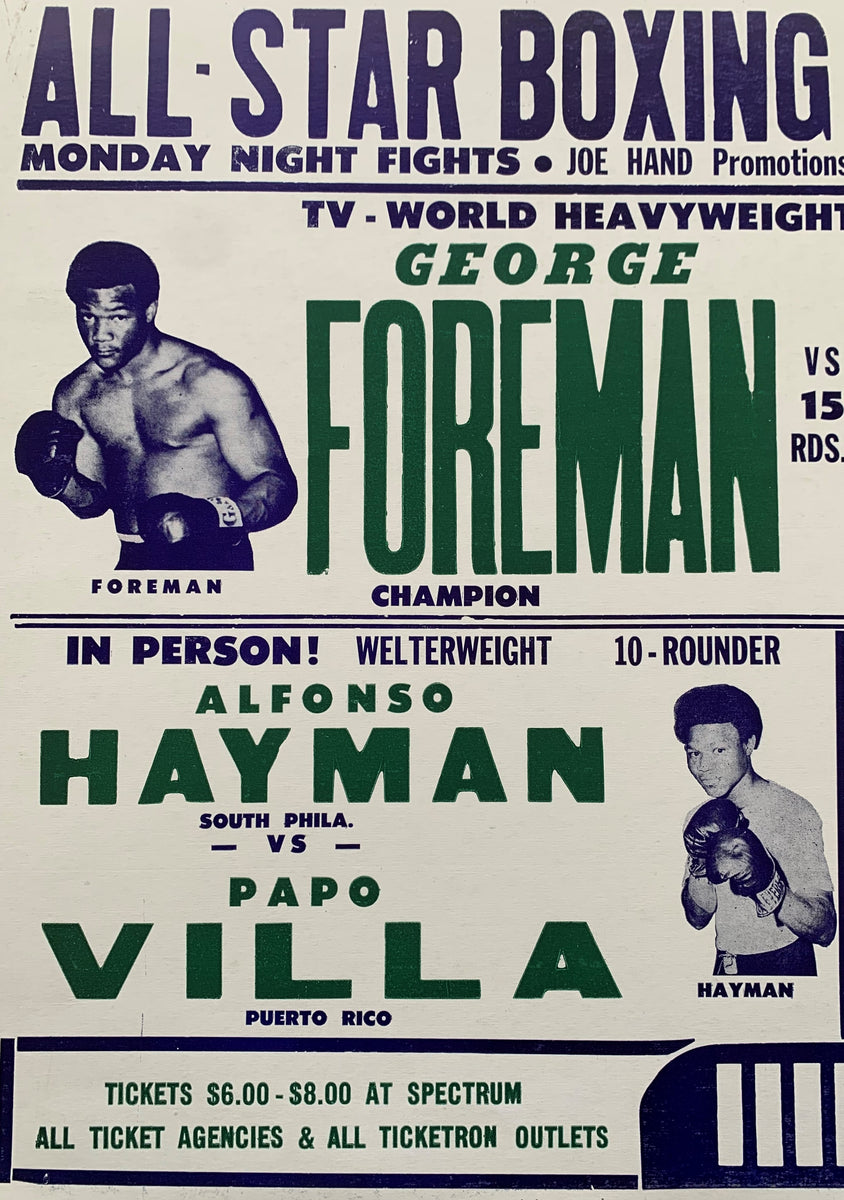The image is a vertically aligned rectangular poster with a light beige background, promoting a boxing event. At the top, in bold navy blue block letters, it reads "ALL-STAR BOXING," followed by "MONDAY NIGHT FIGHTS" in smaller, all caps navy blue text. Below that, a dot precedes "Joe Hand Promotions." A thick horizontal navy blue line separates this section from the rest. 

The next section features an image of a muscular man with black hair and boxing gloves. Underneath the image, in navy blue text, it says "Foreman." To the right of the photo, centered text lists "TV - WORLD HEAVYWEIGHT," followed by "George Foreman Versus 15 RDS" with "champion" underneath. George's name is prominently displayed in tall green letters.

Below this, another section states "IN PERSON!" in navy blue, followed by "Alfonso Heyman" and "South Phila versus Papo via Puerto Rico," with the names in green. An image of Alfonso Heyman with his hands up, positioned to the right, complements this text.

At the bottom, in green text, the poster details ticket prices ranging from $6 to $8, available at Spectrum, all ticket agencies, and All-Ticketron outlets.